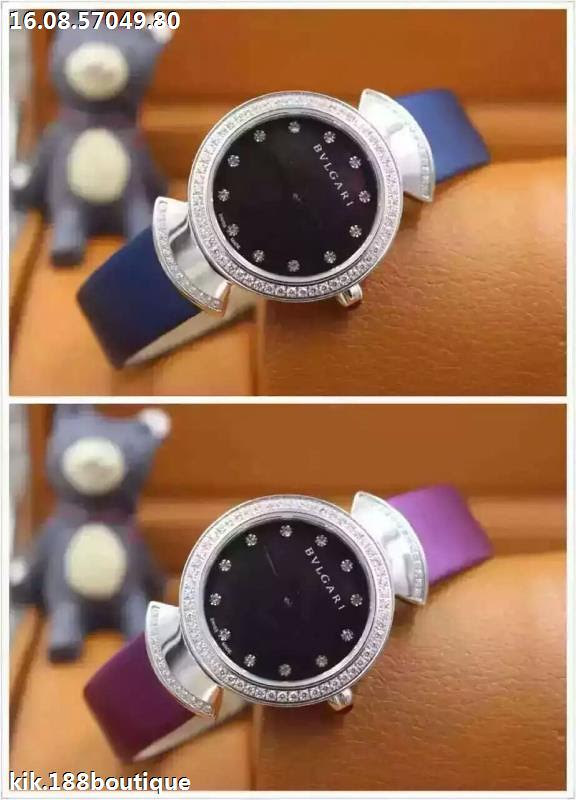This product photograph showcases two nearly identical luxury watches, presented in a two-row format with one photograph above the other. The only distinguishing feature of the watches is the color of their wristbands; the top watch sports a sophisticated navy blue strap, while the bottom watch features a classy pink band. Both timepieces are adorned with elegant silver cases, and the watch faces are framed by a silver ring embedded with sparkling diamonds. The black watch faces prominently display the brand name in silver at the top, and diamonds mark where the hour numbers would typically be. These exquisite watches are set against a tan-colored leather pouch or jewelry box, adding to the luxurious presentation. A charming blue and white teddy bear can be seen on the left side of the image, adding a whimsical touch to the scene.